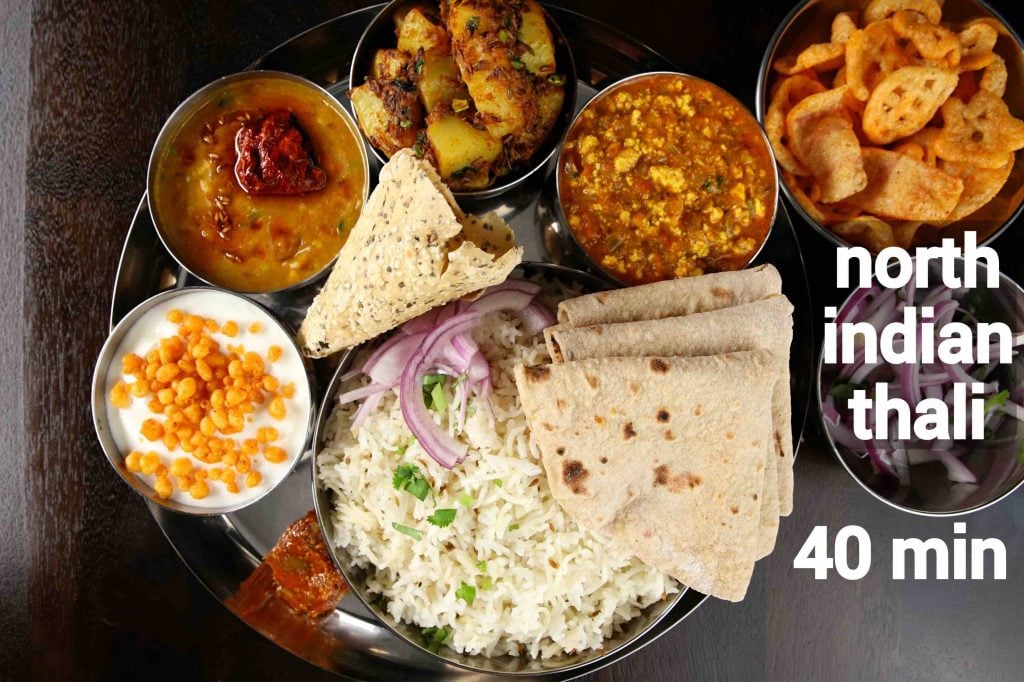This close-up, realistic image depicts an advertisement for a restaurant, showcasing a North Indian Thali. Prominently displayed on a stainless steel serving tray, the Thali features an array of dishes in silver bowls. At the center, the largest bowl contains white rice garnished with purple onions, accompanied by a piece of naan bread. Surrounding the rice are five bowls, each filled with different delicacies: one with a sauce containing corn, a white sauce, a variety of vegetable dishes, and two more soups or sauces. To the right of the tray, two additional bowls can be seen, one containing crisps and the other chopped red onions. The text "North Indian Thali" is displayed in bold white letters at the middle-right part of the image, alongside "40 minutes" also in bold text. The entire presentation is meticulously arranged, emphasizing the vibrant and inviting nature of the food.